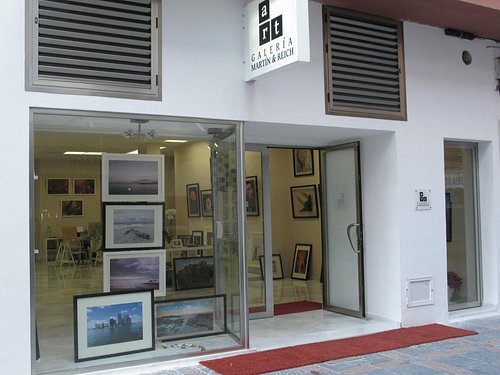The image features the storefront of "Art Galleria Martin and Rausch," characterized by a light-colored stucco exterior and a prominent white sign overhead. The sign creatively displays the word "ART" with the 'A' in a separate block and the 'RT' below. Adjacent to the glass double doors, large metal vents flank the sign, almost as large as the doors themselves. The doors are glass, offering a view into the gallery, which is adorned with numerous framed artworks. To the left of the entrance, the gallery window showcases five framed pieces, stacked vertically with one resting horizontally at the bottom. A bold red doormat lies outside the door, paired with a similar doormat just inside, further inviting visitors into the art-filled interior.